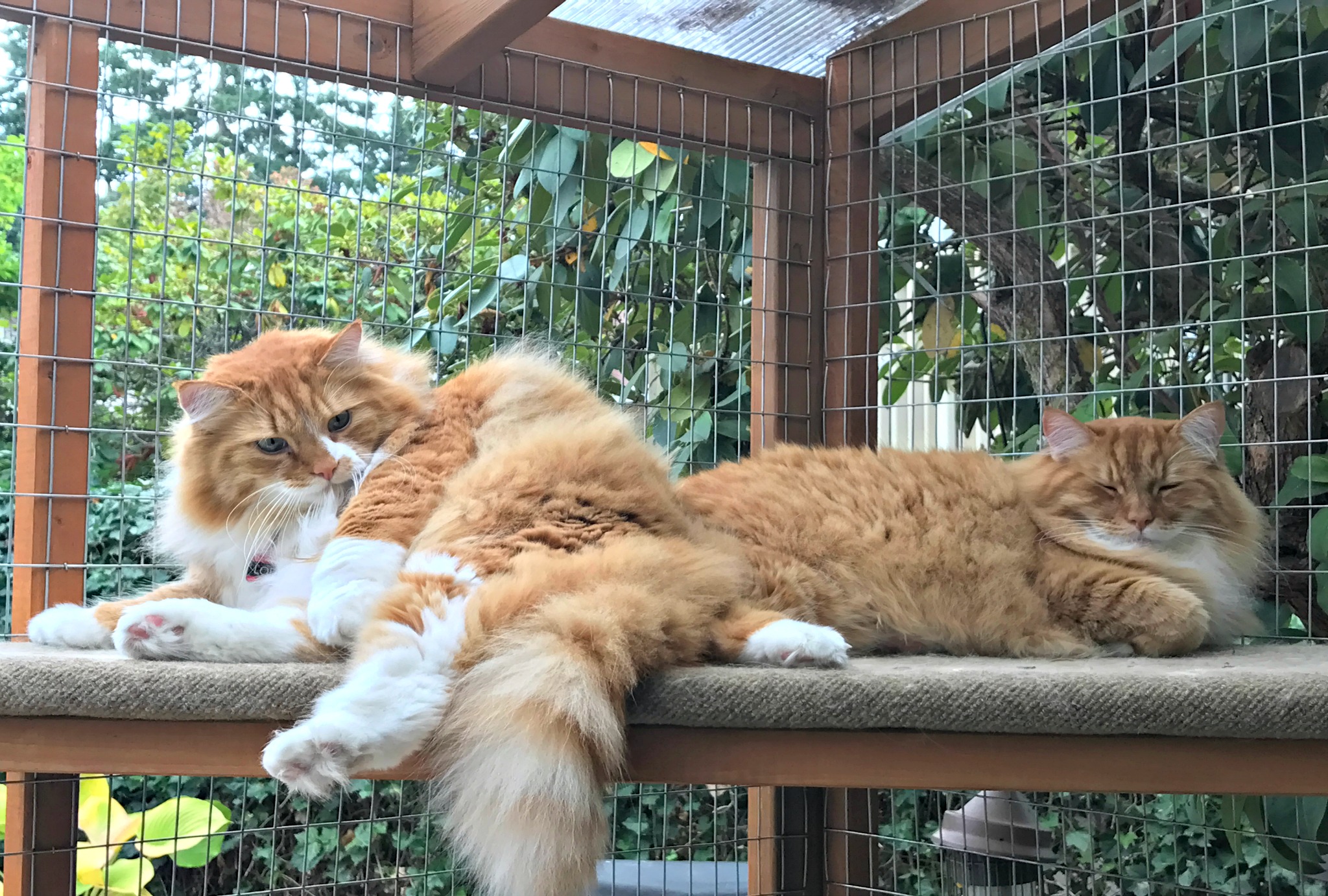In the image, two orange and white cats are lounging on a carpeted shelf within a wooden enclosure secured by chicken wire. The shelf, supported by brown wood beams, is elevated off the ground, giving the cats a cozy perch. The cat on the left, with fluffy fur and bright white markings on its paws, tail, chest, and mouth, appears alert and slightly annoyed as it looks towards the camera. In contrast, the cat on the right, mostly orange except for its white stomach, paws, and inner ears, looks almost asleep. Their heads are positioned at opposite ends of the shelf, creating a balanced yet relaxed scene. Surrounding the enclosure are lush greenery, trees, brush, and some flowers, suggesting a serene, outdoor setting possibly in a backyard. The vibrant daytime light filters through the wire mesh, enhancing the peaceful atmosphere captured in the photograph.